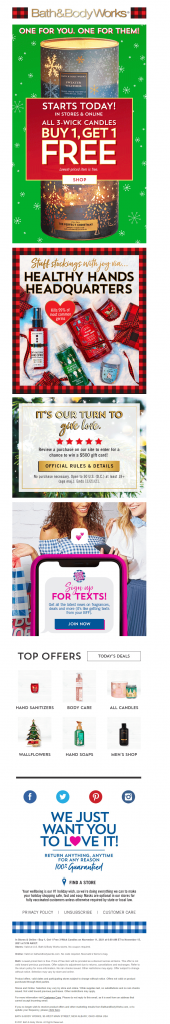The image is a color, portrait-format, digitally produced ad for Bath and Body Works. It seems to be a screenshot that has been squished, making the text and elements appear flattened and somewhat harder to read. At the top, "Bath and Body Works" is prominently displayed. Below, on a green background, it announces the promotion with the text: "One for you, one for them! Starts today. All three-wick candles. Buy one, get one free."

An image of a cylindrical three-wick candle featuring a design of snowflakes and fireworks is shown, exemplifying the offer. Further down, there is an ad titled "Healthy Hands Headquarters," which seems to advertise various moisturizing creams presented in different vials or containers.

Beneath this, there is another segment that is difficult to decipher. Following this, the text "Top Offers" is visible, along with the statement "We just want you to love it." The bottom of the ad contains a large amount of small print, which is typical for disclaimers and additional offer details.